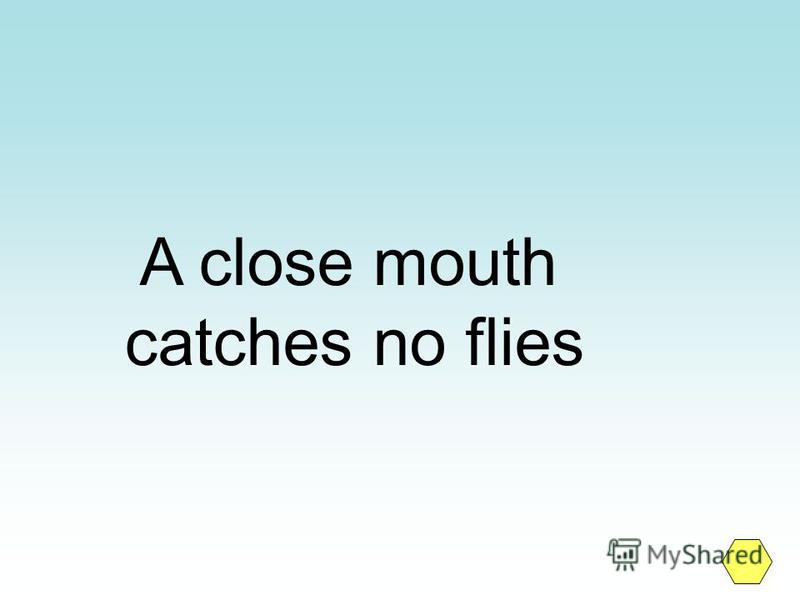The image features a background that starts with a sky blue hue at the top and gradually fades to white at the bottom. In the center, there is a typewritten black text in bold letters that reads, "A closed mouth catches no flies." This phrase is easily visible and stands out prominently against the gradient backdrop. In the bottom right corner, the text "MyShared" appears as a single word in dark gray letters. Overlaid on the last three letters, "RED," is a yellow hexagon with a black outline. This hexagon contains an icon of an easel displaying a flipped-over page with a three-bar graph on it. This detailed composition gives the image a thoughtful and somewhat cryptically insightful appearance.